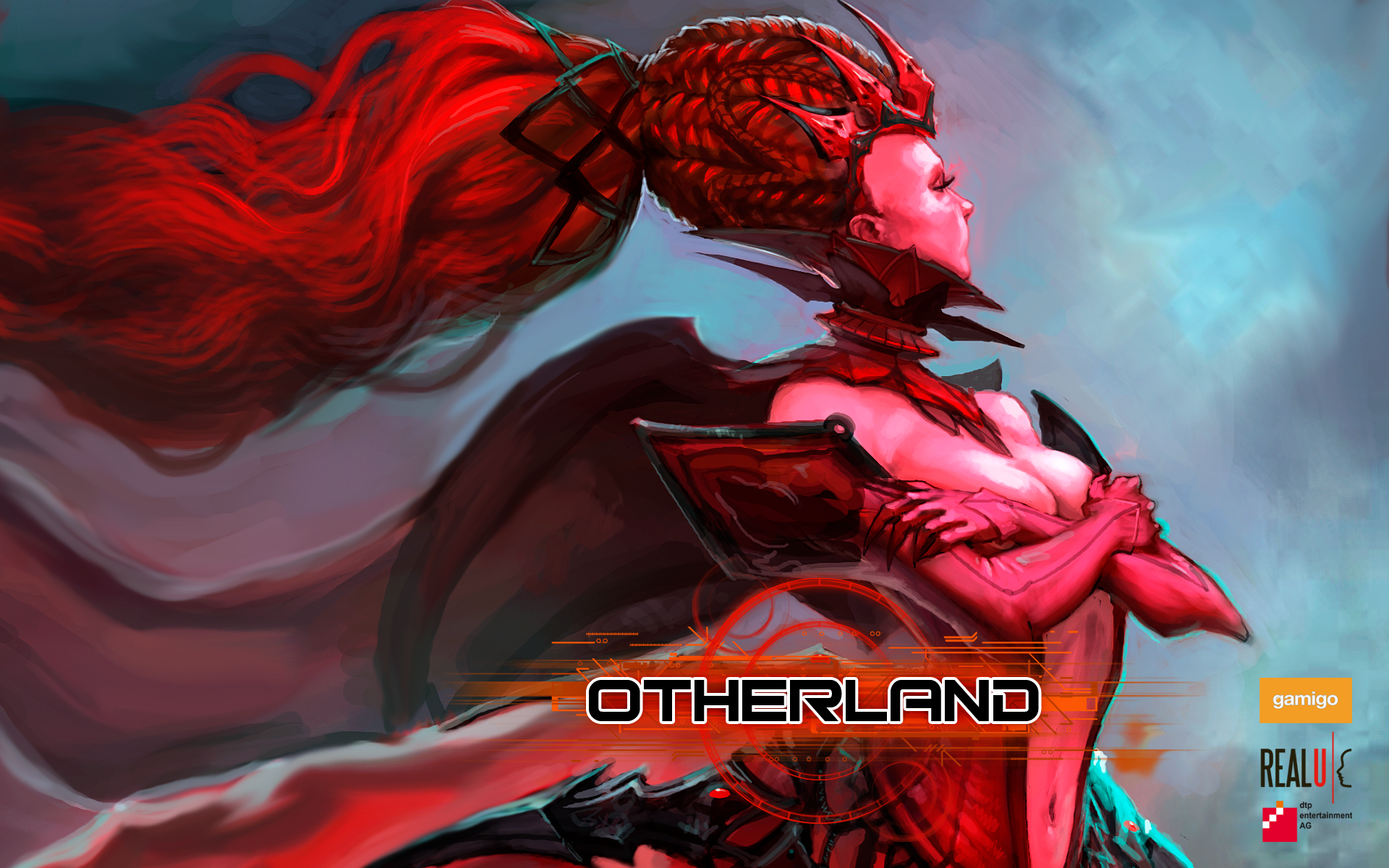The image is a highly detailed, fantasy-themed illustration, likely from a video game or anime movie called "Otherland," with the title prominently displayed in black and white against a circular, target-like logo. The central figure is a mythological, female character with an abundance of elaborate, flowing red hair tied back into intricate braids with a green hair tie. Her skin has a pinkish tint that blends into the overall red palette of her outfit, giving her an almost otherworldly appearance. She wears a striking, strapless, devilish red dress that plunges to her navel, partially revealing her large breasts which are modestly covered by her crossed arms. Her entire body is adorned with red materials, including her gloves that extend to her shoulders and a dramatic neck piece covering her whole neck. The character also appears to wear a crown-like accessory on her head. Her appearance exudes a blend of human and animalistic traits, with claw-like hands and a slightly pinkish skin tone. In the background, the sky is an oil-on-canvas styled mixture of blue and white clouds that accentuates the futuristic and surrealistic elements of the scene. Additional details on the lower part of the image include logos and text such as "Gamigo," "Real You," and an undecipherable block of text adjacent to a small red square with white squares within it, likely indicating the involvement of DIP Entertainment AG in the project.